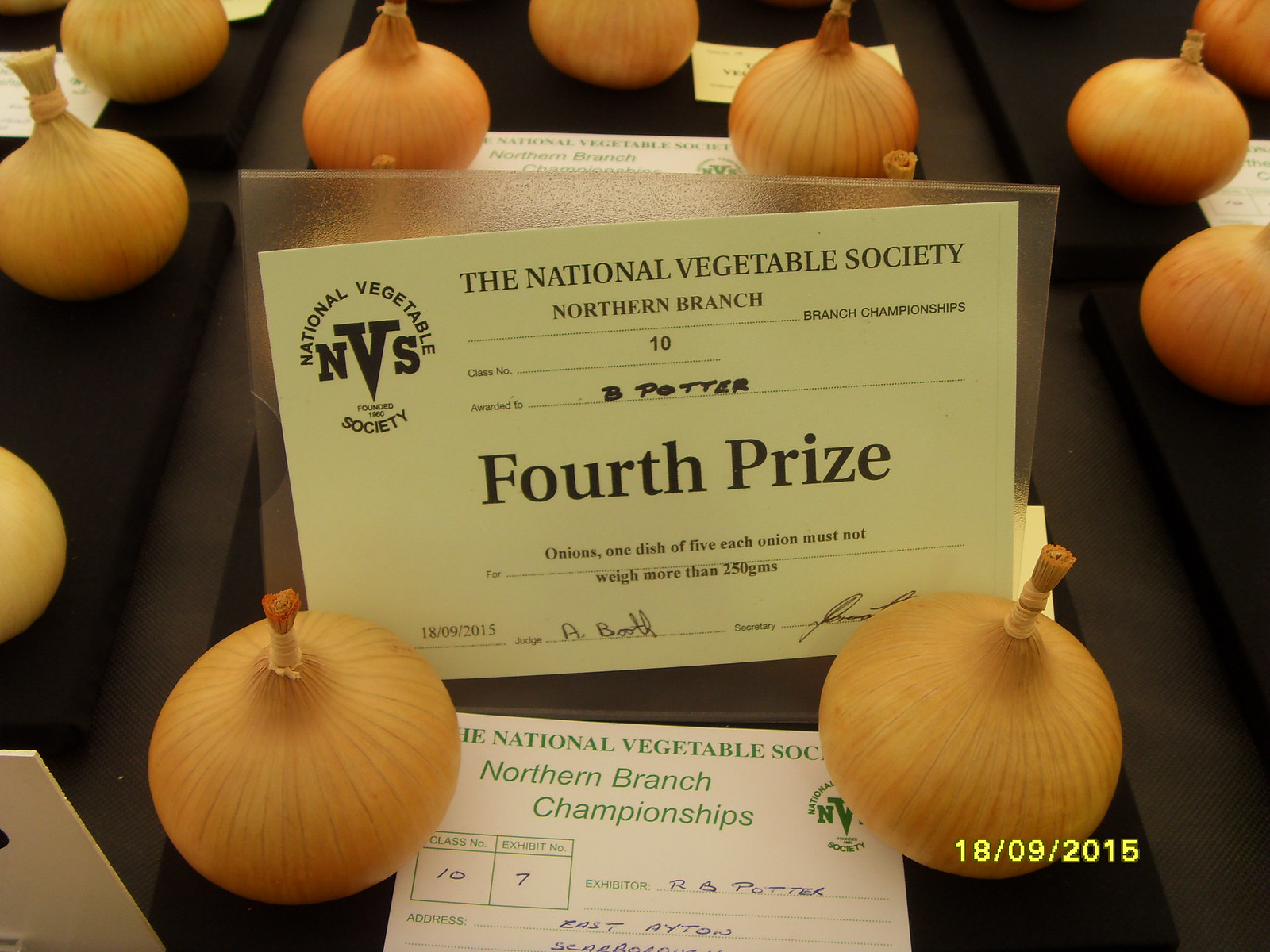The image depicts a competition tabletop showcasing various pairs of onions, all presented on dark-colored brown squares. In the foreground, two perfectly shaped onion bulbs are prominently displayed, having won a certificate from the National Vegetable Society Northern Branch. This certificate, awarded to B. Potter for a fourth-place prize, stipulates that each displayed dish contains five onions weighing no more than 250 grams each. The certificate is signed by Judge P. Booth. Additional pairs of onions with respective cards or forms indicating possible awards are visible in the background. The date "18-09-2015" is noted across the front of the image, highlighting the event's specific timing.